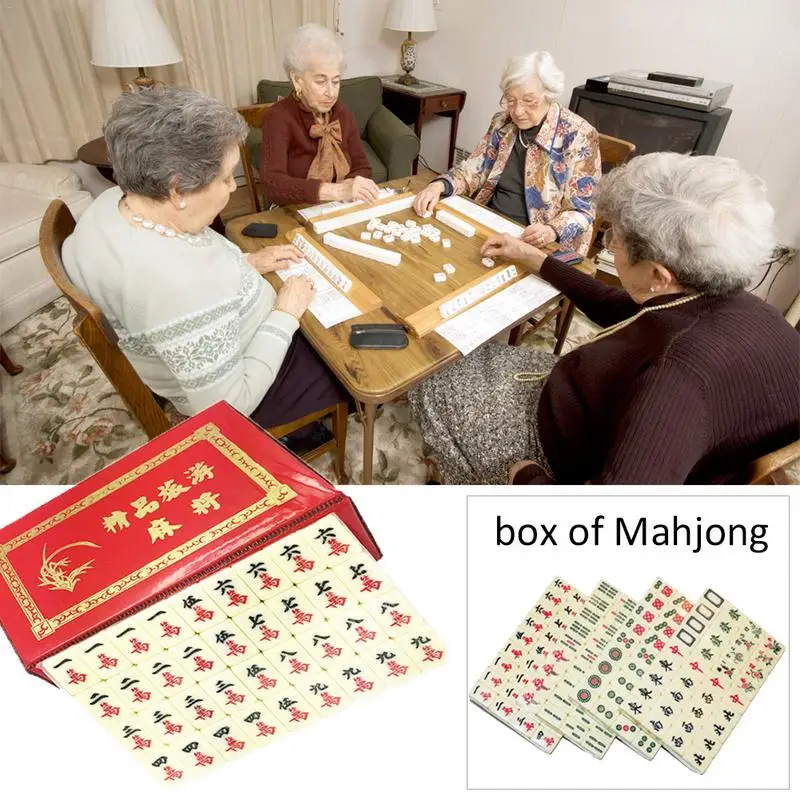The image is divided into two distinct sections. The upper half portrays a cozy living room setting where four elderly women are immersed in a game of Mahjong. They are seated around a wooden table with metal legs, each positioned on wooden chairs. The table's surface is scattered with Mahjong tiles, and each woman has additional tiles in front of them and a piece of paper, presumably for scorekeeping. The room's ambiance is enriched by multiple chairs, an old television with a VCR on top, end tables adorned with lamps, and a carpet underfoot.

In the lower half of the image, a white background showcases several Mahjong-related items. The bottom left features an envelope with a piece of paper bearing Chinese Mandarin characters. The bottom right displays a stack of similar sheets of Mahjong tiles. A prominent red Mahjong box is also highlighted, with the bold text "Box of Mahjong" written in black font beneath it. The image is tinged with hues of white, gray, tan, red, gold, black, and brown, all evenly spaced, creating a well-balanced composition that further emphasizes the theme of a game night in a living room.